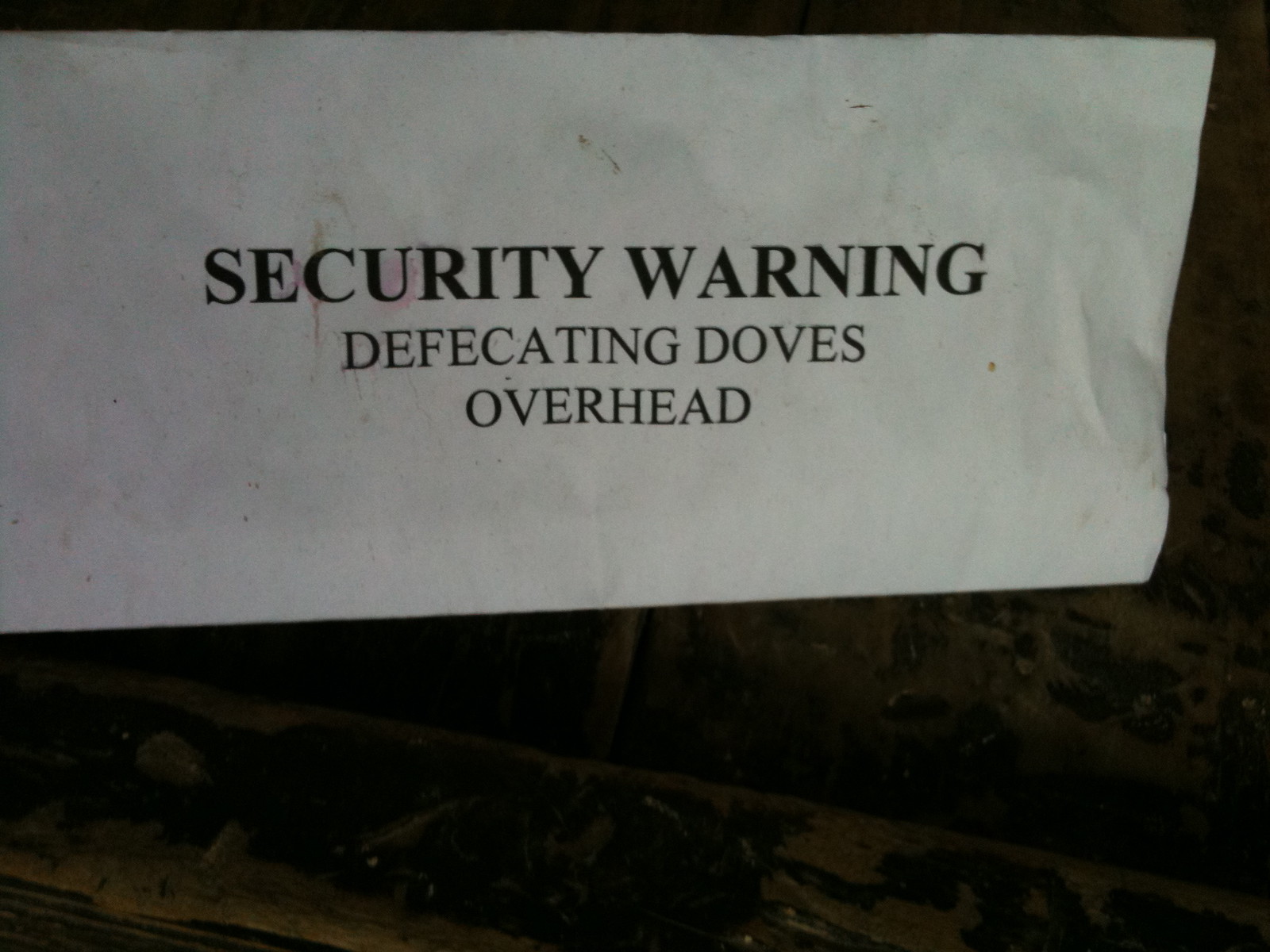The image depicts a satirical security warning sign hanging on a wall in a somewhat dimly lit, outdoor setting. The ground appears dirty, with a mix of colors including white, black, pink, brown, gray, and tan adding to the texture and ambiance. The sign, prominently positioned in the upper part of the image, is a piece of white paper with bold black lettering that reads "Security Warning: Defecating Doves Overhead." This humorous notice warns passersby to be cautious of doves potentially defecating from above. The entire scene suggests both a comedic touch and a practical cautionary message, indicating that the sign is likely meant to provoke a smile while also advising people to be aware of the avian presence overhead.